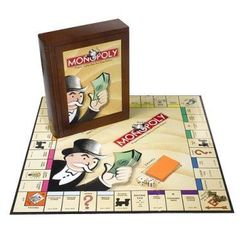In this staged, full-color photograph of the classic board game Monopoly, set against a white background, the focal point is a laid-out Monopoly board taking up the central space. The board features all the familiar elements: various properties, utilities, railroad stations, and the distinctive "Go to Jail" square. The central lower corner prominently displays a larger version of Mr. Moneybags, the iconic Monopoly character, complete with his signature black top hat, white mustache, and a fistful of money. Scattered around the middle of the board are some of the yellow Community Chest and Chance cards. Resting on top of the Monopoly board is a dark brown box, possibly wooden, adorned with a lighter tan Monopoly logo and another image of Mr. Moneybags. Above the logo, there's a red banner with the word "Monopoly." The box's color contrasts nicely with the yellowish background of the board, creating a visually appealing presentation. There are no game pieces or players depicted, emphasizing the pristine and neatly arranged elements prepared for play.